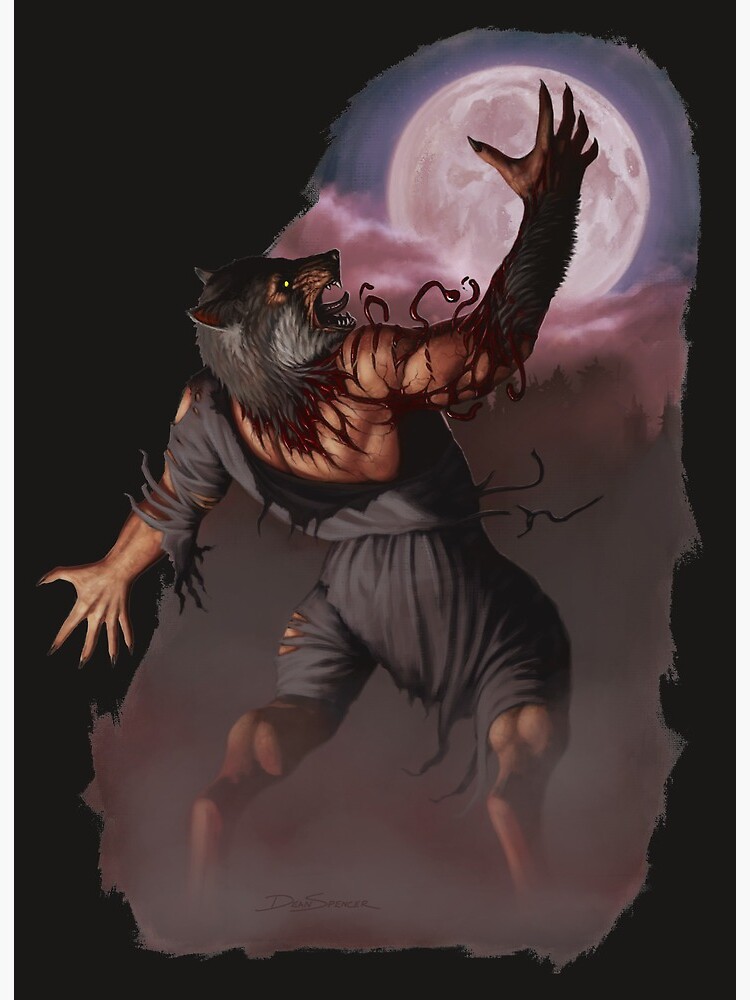The vertical rectangular image vividly portrays a scene of a werewolf mid-transformation. The central figure, a muscular human with the head of a wolf, is viewed from the back, leaping into the air. His face, turned to the right, displays an open, enraged mouth with sharp teeth. The werewolf’s gray, tattered clothes are in disarray, revealing bulging muscles, particularly prominent in his calves. His left arm is stretched behind, showcasing sharp, dark gray or black claws, while his right arm reaches upwards, fingers spread and menacingly clawed. Dark gray hair covers parts of his arms and neck, where blood oozes from fresh claw marks, adding a visceral element to the transformation. The background is a striking blend of black, with a sweeping brush stroke encapsulating a full moon at the top right corner. The moon, a white orb with brown spots, is enveloped in bluish-gray and purplish-red mist, casting a mystical, ominous ambiance over the scene. The werewolf stands on tiptoe, almost blending with the fog and dark atmosphere, creating a dynamic and haunting image of transformation.